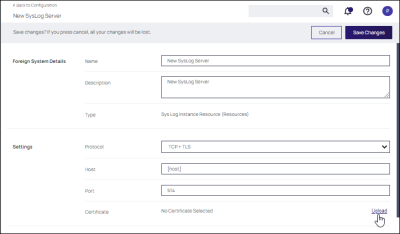The screenshot portrays a minimalist configuration website interface. The layout consists of a new system log server with an option to save changes, warning users that unsaved changes will be lost upon cancellation. The interface includes sections for entering foreign system details like name, description, and type. Despite some complex configurations, it features drop-down menus for selections, showcasing an option for TCP plus TLS. The interface also allows for certificate upload, as indicated by the cursor hovering over the upload button. Text on the page is in a dark purple font, set against a primarily white background, contributing to the straightforward but somewhat indistinct visual presentation.